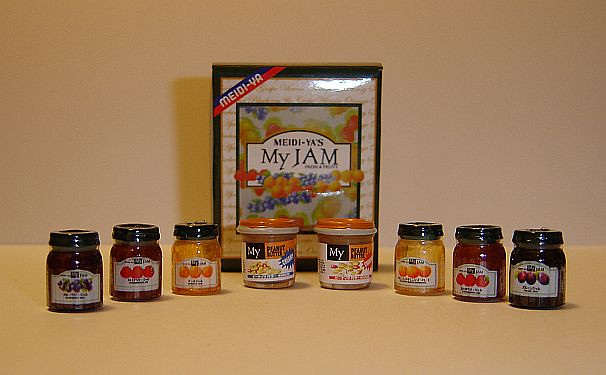This image captures an arrangement of eight jars set against a light brown, peachy beige surface. The background showcases a cream-colored wall. At the back, there's a black-framed image that resembles an advertisement or box cover with the words "Medi Yass, My Jam" prominently displayed above depictions of various fruits such as grapes, peaches, raspberries, and strawberries.

In the foreground, the jars are arranged in a slight crescent shape, curving away from the viewer. Six of these small jars contain different flavors of jam and are equipped with black twist-off lids. The jam flavors identifiable from the visible fruit illustrations include grape, raspberry, peach, strawberry, and possibly plum or blueberry. Interspersed among them, the two center jars are distinct with orange tops and are labeled as peanut butter—one being cashew, while the other flavor is obscured.

This detailed setup highlights a curated collection of preserves and peanut butters, framed by an advertisement-like background image, suggesting a vibrant and artisanal approach to common breakfast spreads.